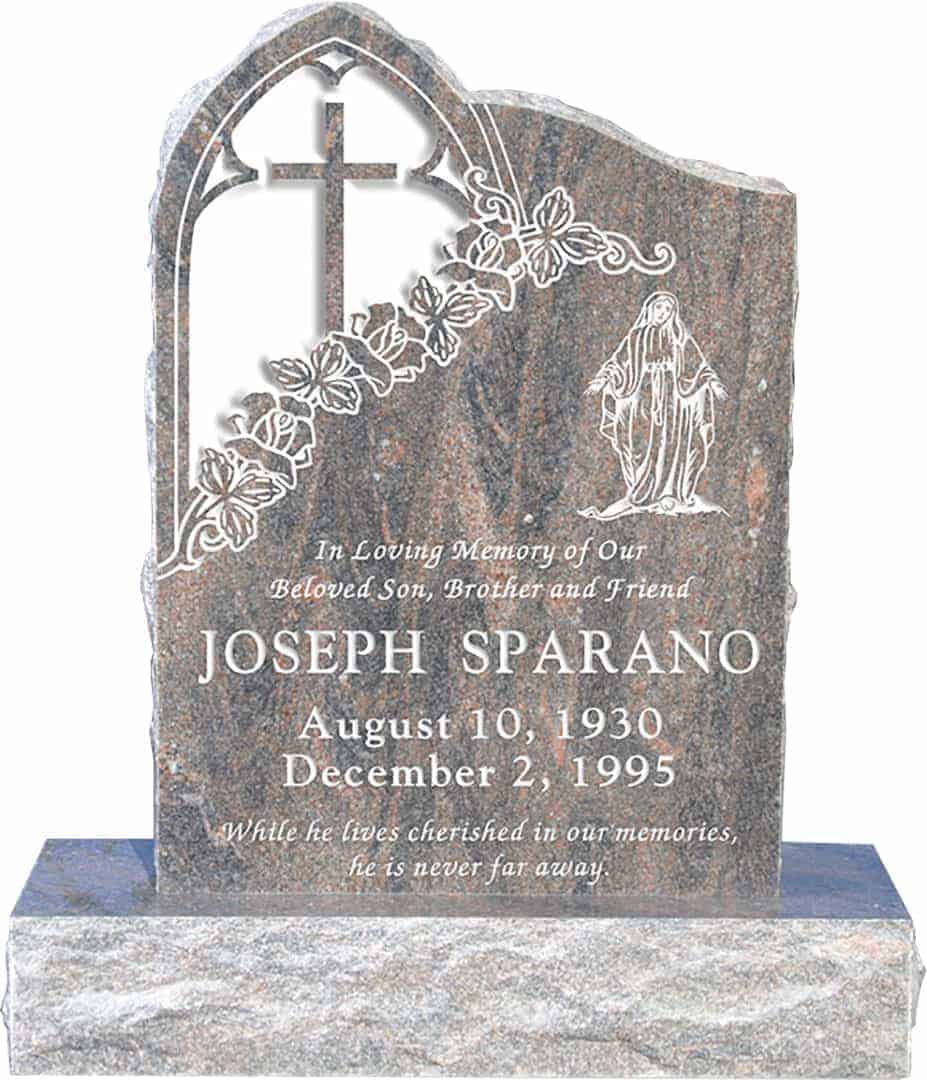This black-and-white photograph features a dark brown granite tombstone, mounted on a cement or granite pedestal. The tombstone's text, inscribed in white, reads: "In loving memory of our beloved son, brother, and friend, Joseph Sperano, August 10, 1930 - December 2, 1995. While he lives, cherished in our memories, he is never far away." The top left corner of the tombstone showcases an engraved crucifix adorned with a floral and leaf design. On the upper right side, a white silhouette of the Blessed Mother, likely the Virgin Mary, is prominently displayed. The meticulous details and heartfelt inscriptions pay tribute to Joseph Sperano, preserving his memory in a somber, elegant monument.